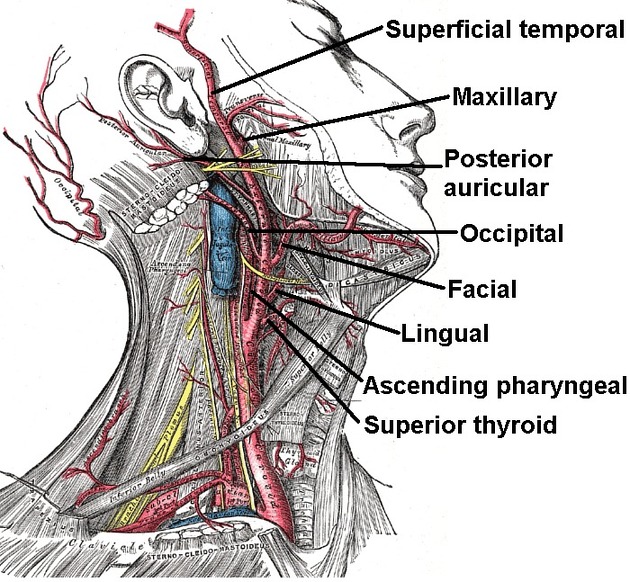This anatomical diagram, set against a solid white background, depicts the side view of a human head and neck, focusing on the circulatory system. The head is slightly tilted backward, with the nose pointing towards the top right. The diagram predominantly features red veins, which are meticulously labeled with black text. At the top, the superficial temporal vein extends upward, followed by the maxillary vein situated lower on the face. The posterior auricular vein is located near the bottom behind the ear, and the occipital vein is positioned at the back of the head. Further details include the facial vein, slightly under other layers, and the lingual vein. Completing the diagram, the ascending pharyngeal and superior thyroid veins are also labeled, providing a comprehensive overview of the primary veins in this head and neck region.